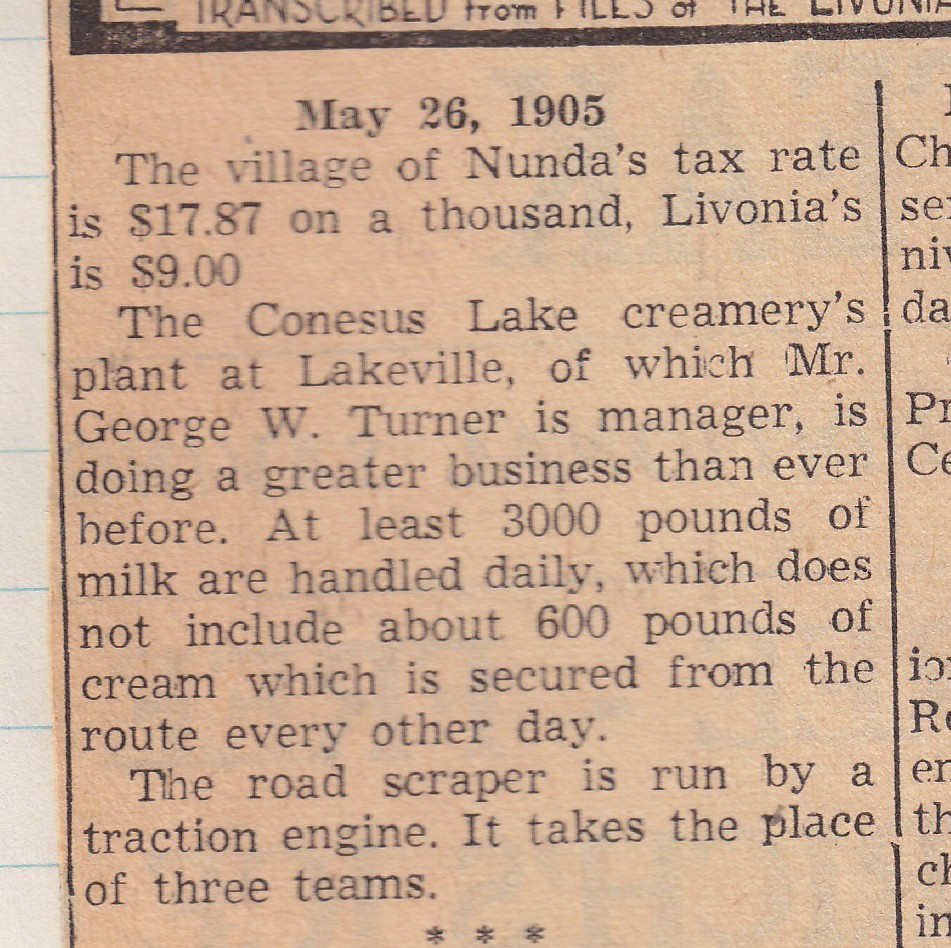This image depicts a discolored and aged newspaper article dated May 26, 1905, carefully cut out and laid on white ruled paper with faint blue lines. The paper has a pinkish or peach hue, typical of its age, with clear black print. The article details various local updates, mentioning that the tax rate in the village of Nunda is $17.87 per $1,000, whereas Livonia's tax rate is $9. A significant portion of the article discusses the Conesus Lake Creamery plant at Lakeville, managed by Mr. George W. Turner, which handles over 3,000 pounds of milk daily and about 600 pounds of cream every other day. It also notes the use of a traction engine to operate the road scraper, replacing the need for three teams. The article's content is partially obscured by a black vertical line on the right side and ends with three asterisk signs at the bottom.